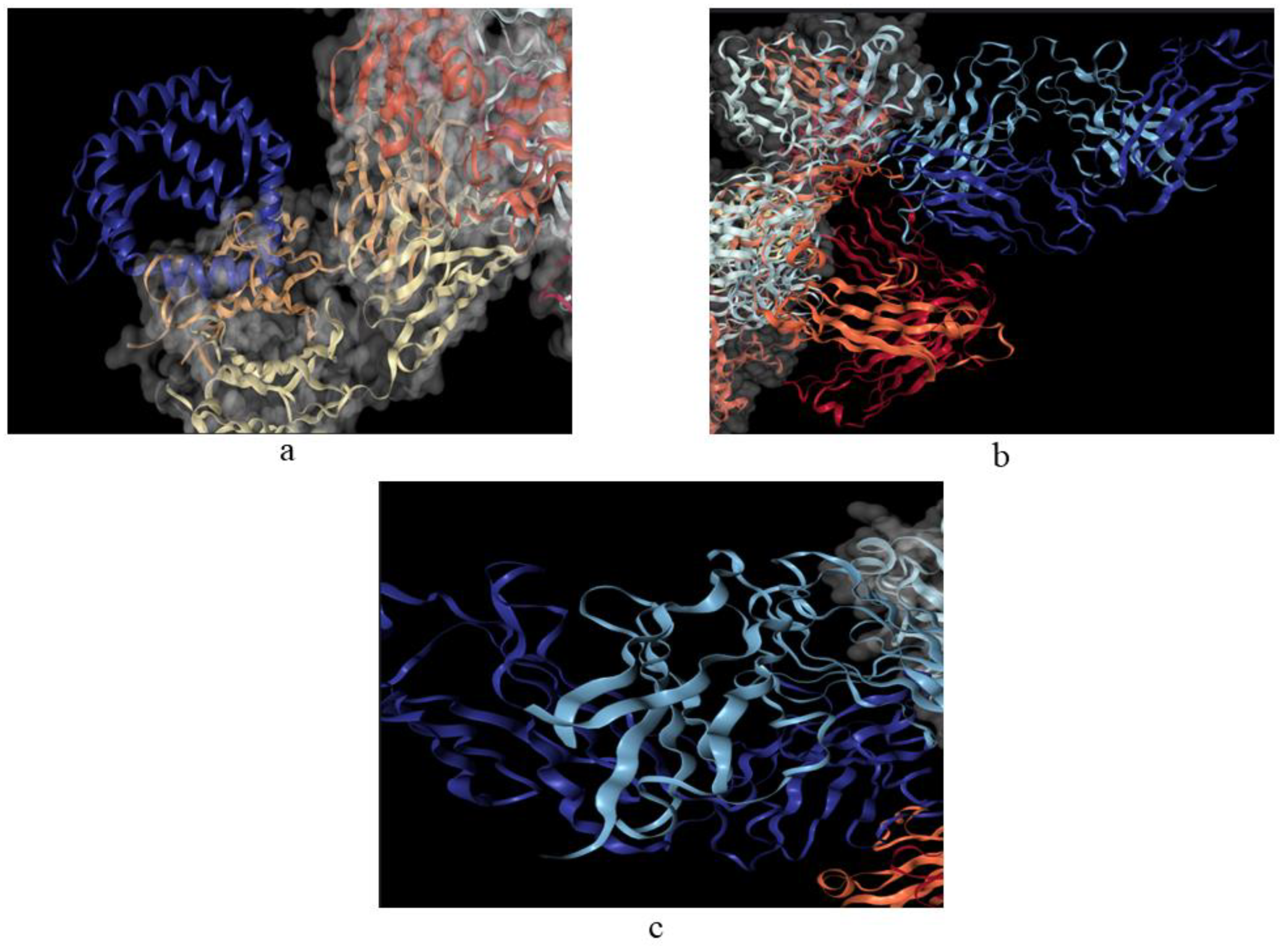The image showcases a triptych of three photographs labeled A, B, and C against a jet-black background. The top row features images A (left) and B (right), while the bottom row is labeled C. Each photograph displays an intricate array of colorful ribbons, including shades of blue, orange, yellow, red, and grayish-white, with a smoky, ethereal quality entwined throughout. In image A, predominantly dark gray, yellow, blue, and red ribbons twist and interweave in a seemingly random but visually arresting composition. Image B highlights swirling strands of blue, orange, grayish-white, and red, evocative of flowing hair or smoke drifting to the side. Finally, image C, at the bottom, focuses on various shades of blue, with dark and light blue ribbons dominating the scene, complemented by hints of red-orange and gray in the top and bottom corners. The ribbons in all three images appear to coil and flow freely, creating a dynamic and almost chaotic visual effect.